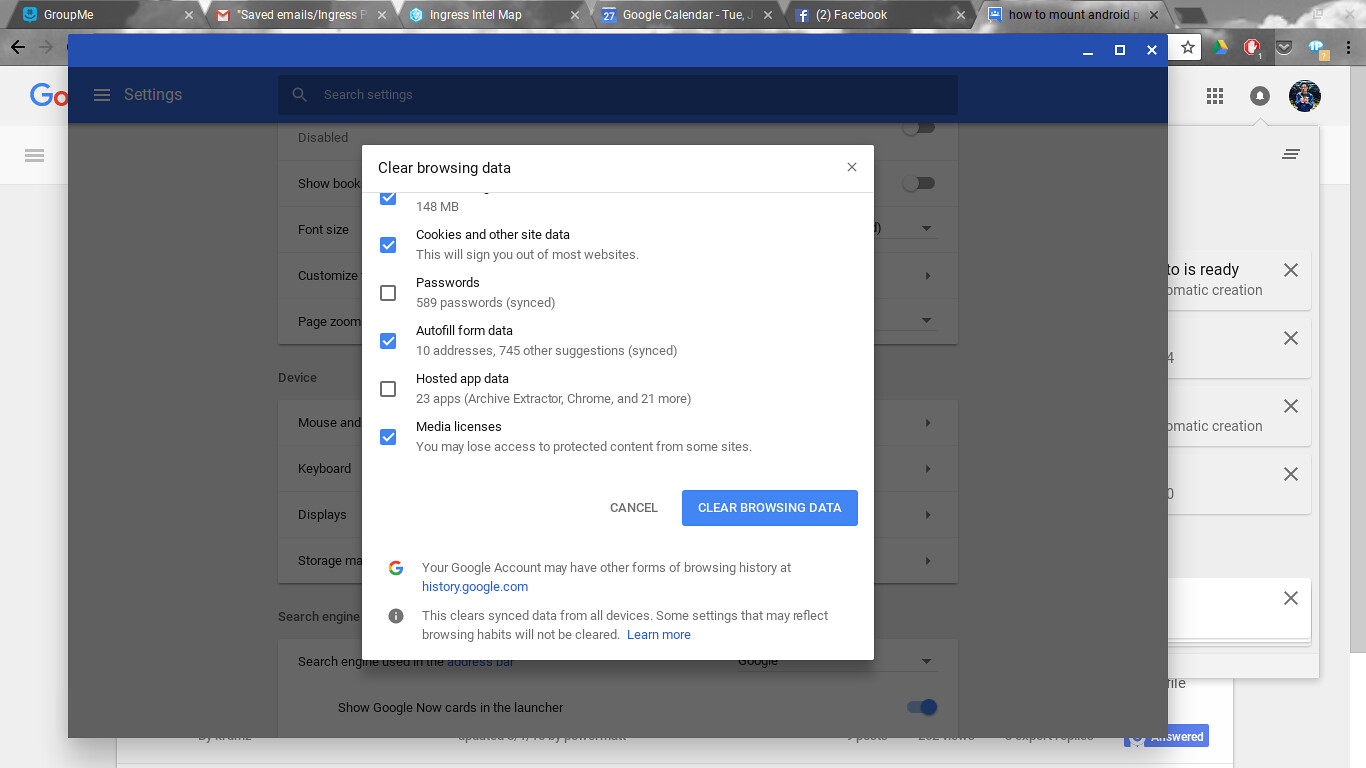The image depicts a computer screenshot in a rectangular format with the longer side stretching from left to right. The primary focus is a Google Chrome browser window with six visible tabs. Overlaying this is a semi-transparent, grayed-out screen featuring a central white dialog box titled "Clear browsing data." Within this dialog box, the text is rendered in black, listing options with checkboxes and accompanied by a large blue button labeled "Clear Data" near the bottom-right corner.

The checkboxes are filled with blue, each containing a white checkmark. The options with checkmarks that are clearly visibile include:
- Cookies and other site data
- Autofill form data
- Media licenses

In the background, under the white overlay, the edges of the main browser window are slightly obscured but visibly grayed-out. The browser itself shows a blue border. The open Chrome tabs are labeled: "How to mount Android," "Facebook," "Google Calendar," "Ingress Intel Map," "Saved Email Ingress," and "Group Me."